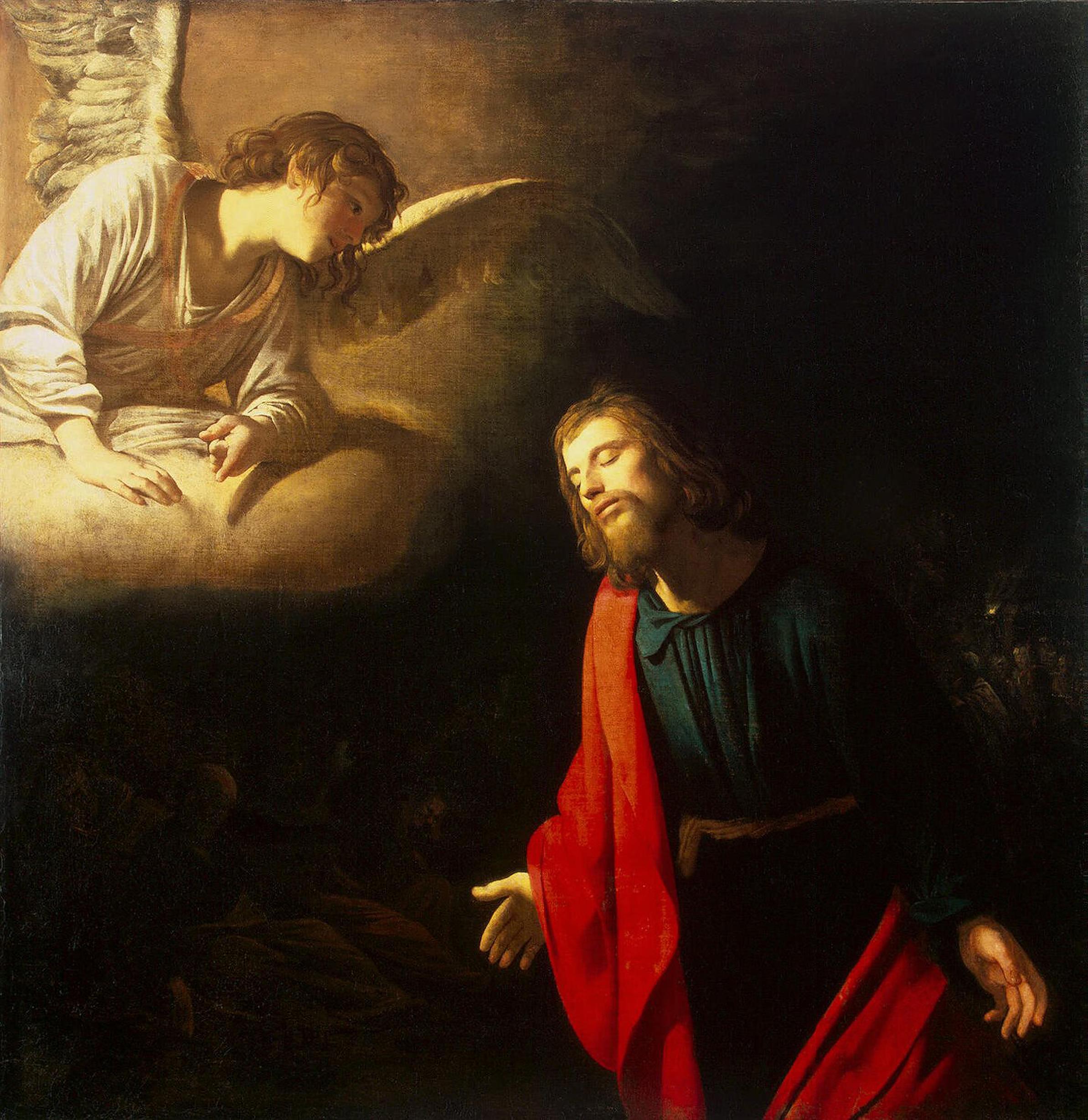This painting, reminiscent of the old masters' style, depicts a deeply spiritual and somewhat somber scene characterized by its dark and cavernous background, where shadowy human forms blend into the blackness. Dominating the lower right corner is Jesus Christ, bearing long brown hair and a goatee, clothed in a dark blue robe with a red shawl draped over his right shoulder and tied around his waist. His eyes are closed, and his peaceful demeanor is emphasized by his outstretched hands, palms upturned, bathing in a soft yellow light that illuminates his face and hands. In the upper left corner, an angel, or cherub, sits atop a cloud-like cushion with white wings extending from their back. The angel, with blue curly hair and a white robe, adorned with a gold ribbon at the bottom, gazes down at Jesus with an ethereal expression. The overall atmosphere is one of reflection and divine presence, tinged with a slight sense of mystery and the supernatural due to the dim, shadowed surroundings.